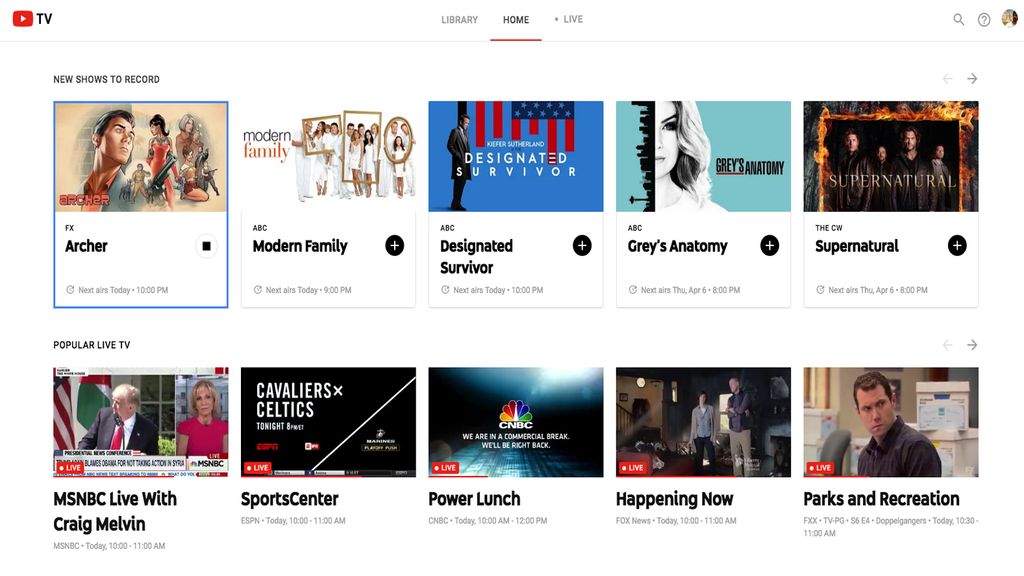This image depicts the interface of YouTube TV. In the upper left-hand corner, there is the recognizable red YouTube logo - a red box with a white play button inside it, followed by the word "TV" in black. Spanning the top of the screen are menu options labeled "Library," "Home," and "Live," with "Home" currently selected. 

On the top-right corner, there are three icons: a magnifying glass representing the search function, a question mark encased in a circle for help, and a user profile picture within a red circle. Below these elements is a section titled "New Shows to Record," featuring a horizontal row of thumbnails for five different shows: "Archer," "Modern Family," "Designated Survivor," "Grey's Anatomy," and "Supernatural." 

Underneath this, there is another section labeled "Popular TV," which showcases a variety of programs including "MSNBC Live with Craig Melvin," a sports event titled "Cavaliers and Celtics" from SportsCenter, "Our Lunch," "Happening Now," and the comedy series "Parks and Recreation."